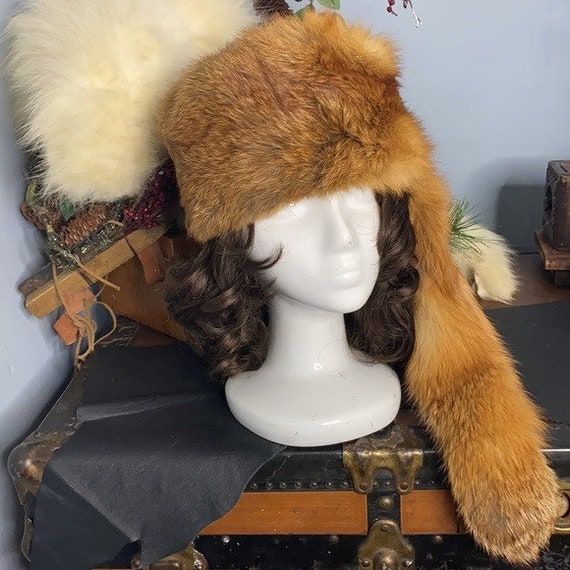This is a detailed, color photograph featuring a white mannequin head adorned with a layered arrangement of headpieces. The mannequin, situated atop an antique-style black footlocker chest with gold metal fixtures and wooden accents, sports a shoulder-length, curly brunette wig. Atop the wig is a large, light brown fur cap resembling fox fur, with feathers peeking out from behind it. To the left of the mannequin head, additional fur items and another wooden object can be observed, contributing to an overall aesthetic reminiscent of a retro clothing store or an antique rummage sale. The setup evokes a sense of nostalgia and old-school charm.